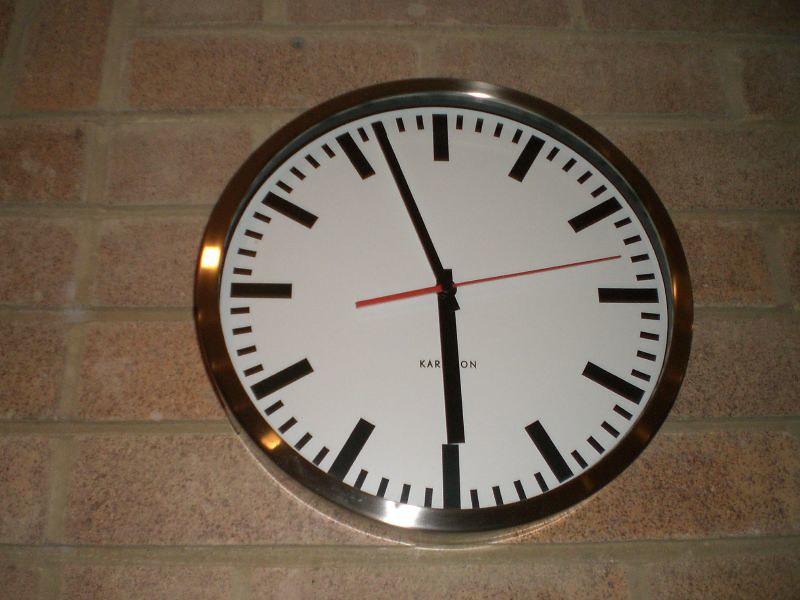A red brick wall serves as the backdrop for a metal-rimmed, flat wall clock without any numbers. The clock, which has a brown metallic rim and black minute and hour hands, features dashes to indicate time, with larger dashes marking the positions where numbers commonly would be. A red second hand is currently pointing at the 14-second mark, while the time displayed is approximately 5:57. This minimalist clock is mounted directly onto the textured brick, creating a striking visual contrast.